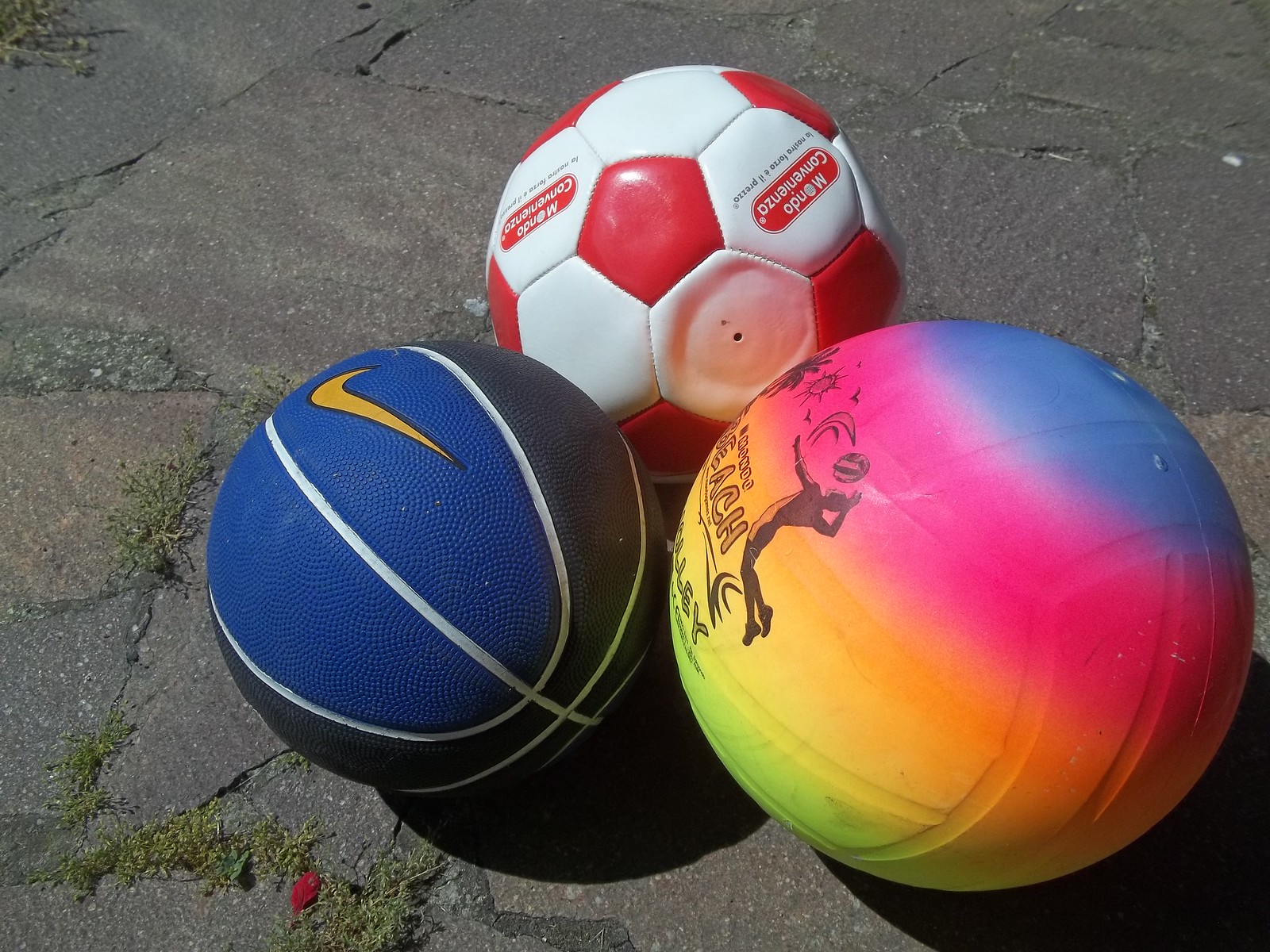In the image, three vividly colored balls are positioned on a grey cement driveway peppered with green moss and some scattered weeds sprouting through the cracks. The ball on the left is a basketball featuring bold royal blue and black stripes, adorned with a yellow Nike swoosh in the center. Towards the back of the image sits a red and white soccer ball, bearing the label "Mondo Cavencia," appearing slightly deflated and in need of air. In the foreground, you see a vibrant volleyball with a top section colored blue, a middle ring in pink, and a bottom section transitioning from light orange to a bright green. This volleyball also features an image of a person in black, captured mid-air in an attempt to spike the ball. The cracked cement and sporadic patches of moss add a rustic charm to the setting, complemented by the presence of a small red flower.